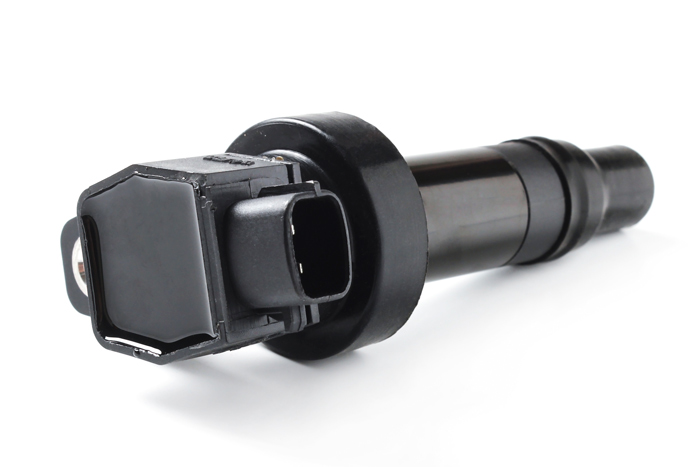The photograph captures a black, likely metallic, object lying on its side against a white background, the stark contrast accentuating its intricate features. The object appears to combine elements of plumbing, photo equipment, or possibly an electrical component. Starting from the right, a small black cylinder is nested within a larger one, with a noticeable seal wrapped around it. This assembly continues into a slimmer cylinder that angles slightly towards the camera on the left. This sequence culminates in a circular disc reminiscent of a hockey puck, also black. Atop this disc sits a not-quite-square connector or sensor, featuring an opening with two prongs, suggesting it serves as an adapter or charger. The top of this component, which is a lighter black or dark gray, bears raised, albeit unreadable, lettering. The total length of the object is estimated to be around six inches, its sleek, jet black metallic surface adding to its enigmatic yet functional appearance.